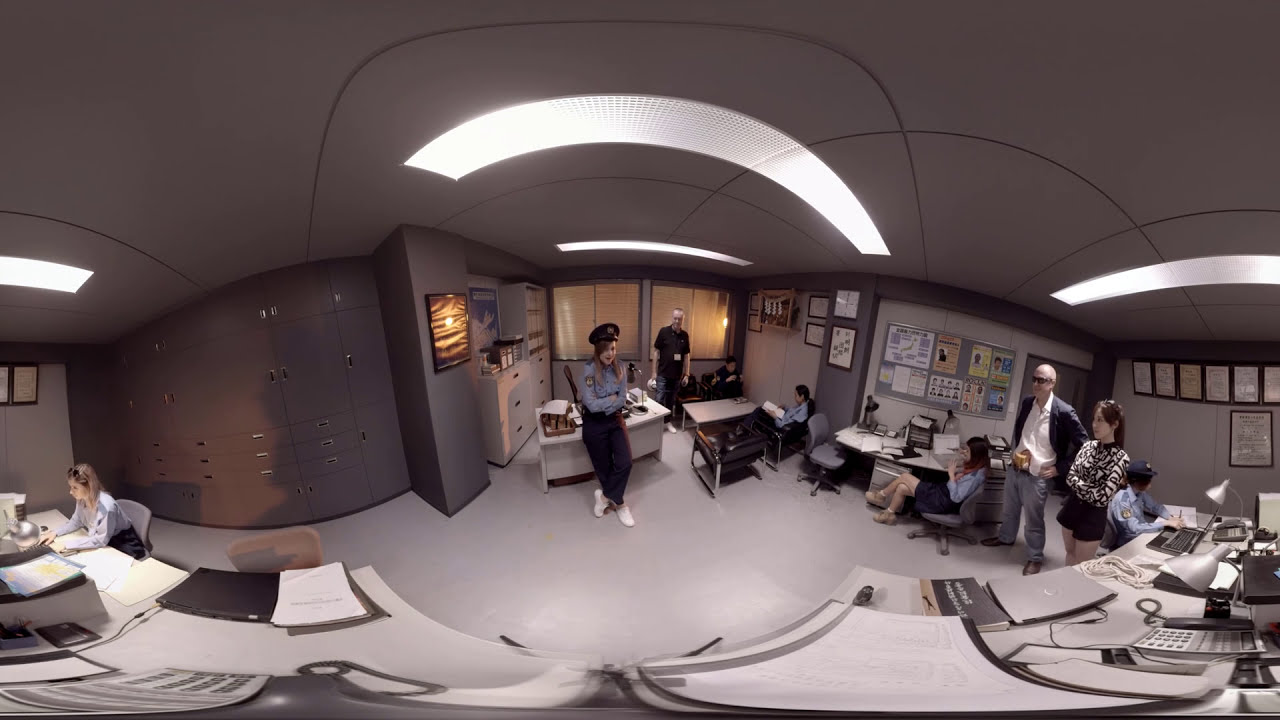The image is a panoramic fisheye 360 view of what appears to be an office setting, possibly a police station. At the center of the image, drawing immediate attention, is a policewoman dressed in black pants, a blue long-sleeve shirt, and a hat, possibly indicating her role or rank. She stands confidently, smiling at the camera. The environment is characterized by white tiled floors, gray walls, and a ceiling fitted with curved fluorescent lights that dimly illuminate the room. 

Several other individuals are dispersed throughout the space, engaged in various activities. On the left side of the image, a woman with a ponytail, possibly another officer, is seen sitting at a desk, either writing on a notepad or reading a book. Nearby, another woman with sunglasses perched on her head types on a keyboard. Behind the central policewoman, a man in a short-sleeved black shirt and jeans stands observing the scene. 

The right side of the room features a group of people, some standing and others seated, suggesting diverse interactions and possibly civilian presence. A man in jeans, a white shirt, and a brown or blue jacket stands out among them. Another individual in black shorts and a white and black print long-sleeved top, also with hair in a ponytail, stands near someone in a blue outfit, busy typing on a laptop. 

The back wall is lined with dark gray lockers or built-in filing cabinets, adding to the structured office environment. Papers, keyboards, and other office supplies are scattered across multiple desks, emphasizing the bustling yet orderly atmosphere of what is likely a public service office, where both officers and civilians converge.